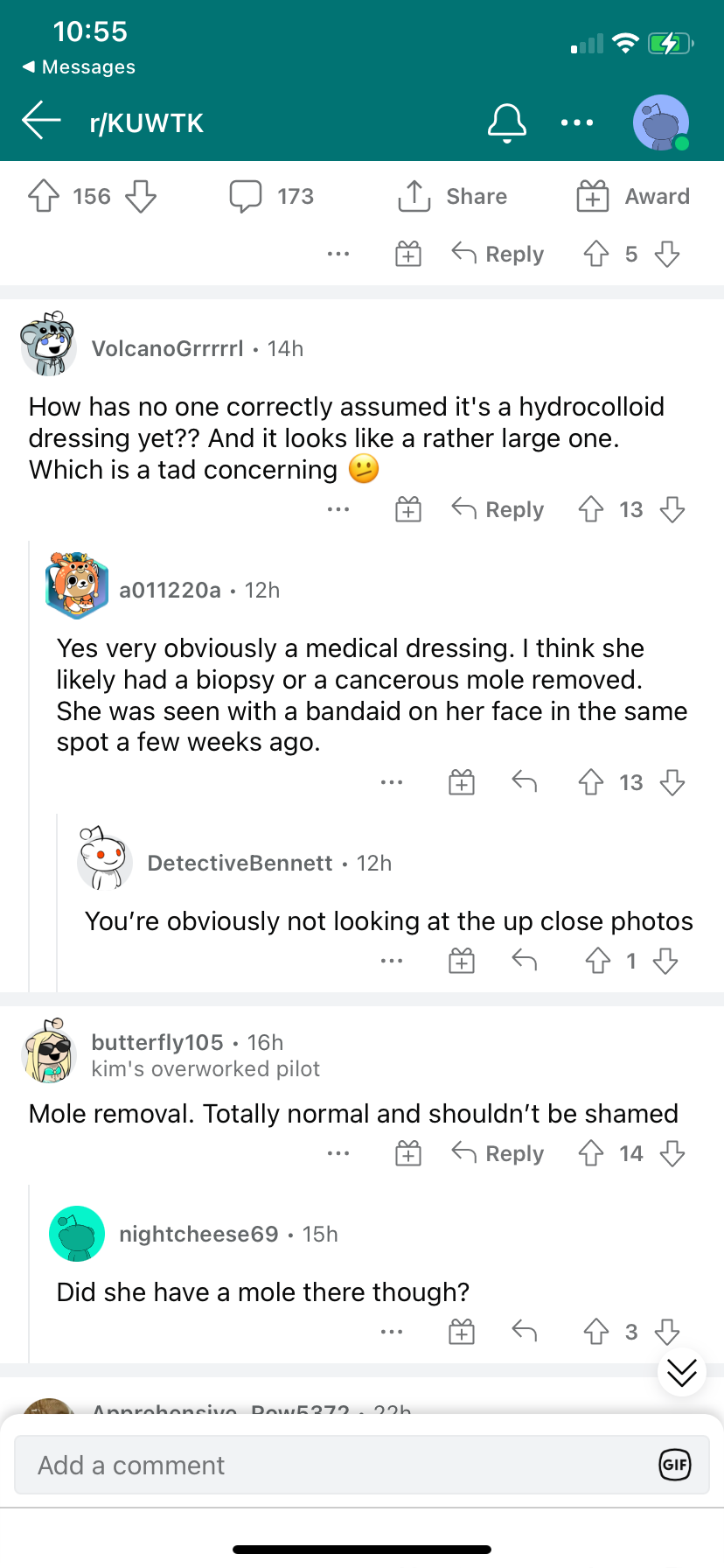A vibrant, color portrait mode screenshot of a smartphone taken at 10:55 AM, showing the device with one out of four bars of reception and approximately 90% battery life. The user is browsing Reddit, specifically on the subreddit r/KUWTK, a community dedicated to discussing "Keeping Up with the Kardashians." The screenshot captures a post with 156 upvotes, 173 comments, and options for sharing and awarding. The user has scrolled down to the comments section, where discussions revolve around a hydrocolloid dressing. The top comment by "volcano_girl" questions why no one has correctly identified the item as a hydrocolloid dressing, noting its large size and expressing some concern. Following this, another user confirms it is indeed a medical dressing, with the conversation continuing further down the thread.